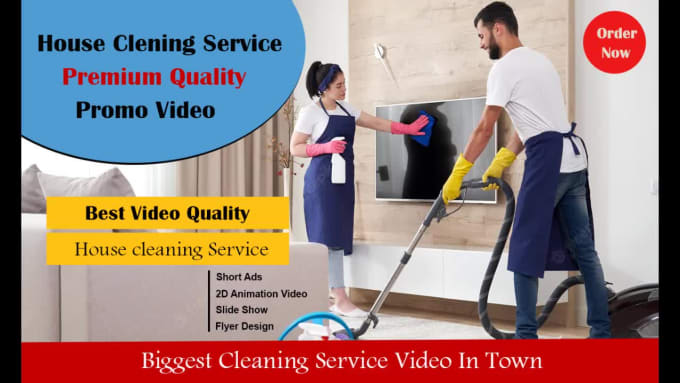This advertisement for a house cleaning service features a high-quality promotional video set in a neutral-toned living room. The top left corner contains a blue oval with a text error— the phrase "House Cleaning Service" is missing the 'A' in "Cleaning." Beneath this, "Premium Quality" is displayed in red, followed by "Promo Video" in black. In the background, a woman with brown hair tied in a ponytail is wearing a white t-shirt, jeans, and a navy blue apron as she cleans a television with a blue rag and a white spray bottle. She dons hot pink gloves reaching her forearms. To her right, a man with dark brown hair in a white t-shirt, jeans, and a waist-length blue apron is vacuuming or steam cleaning the carpet, wearing yellow forearm gloves. The top right corner features a red circle with "Order Now" in white text, while the bottom part of the image highlights various promotional elements, including yellow bars with "Best Video Quality" and "House Cleaning Service," and a red running banner stating "Biggest Cleaning Service Video in Town" in white.